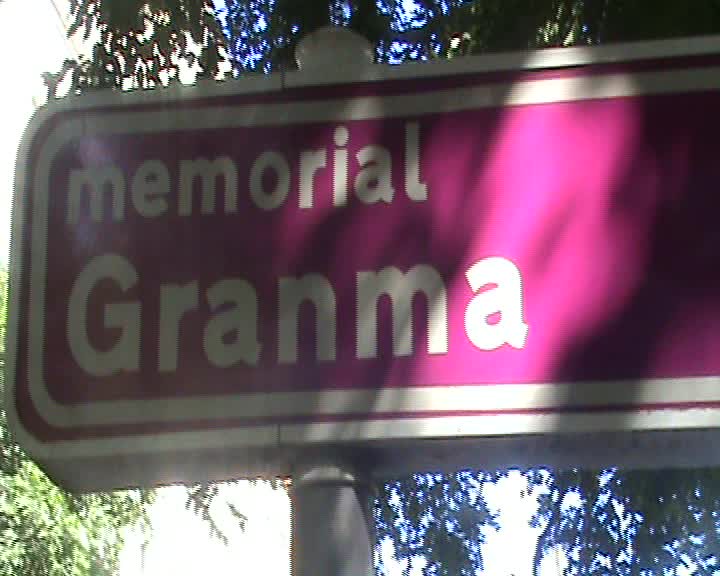The image showcases a white sign with a noticeable offset signpost, implying the potential presence of another post at the unseen right end. The sign features a dual white border, with a slim purple line nestled between the outer and inner white edges. Inside the bordered area, the sign displays a flat, purple background. Bold, white text in large letters reads "MEMORIAL GRANDMA," with "GRANDMA" uniquely spelled as "G-R-A-N-M-A." The scene behind the sign includes a bright, daytime sky and dense, green tree foliage, giving a natural, vibrant backdrop.